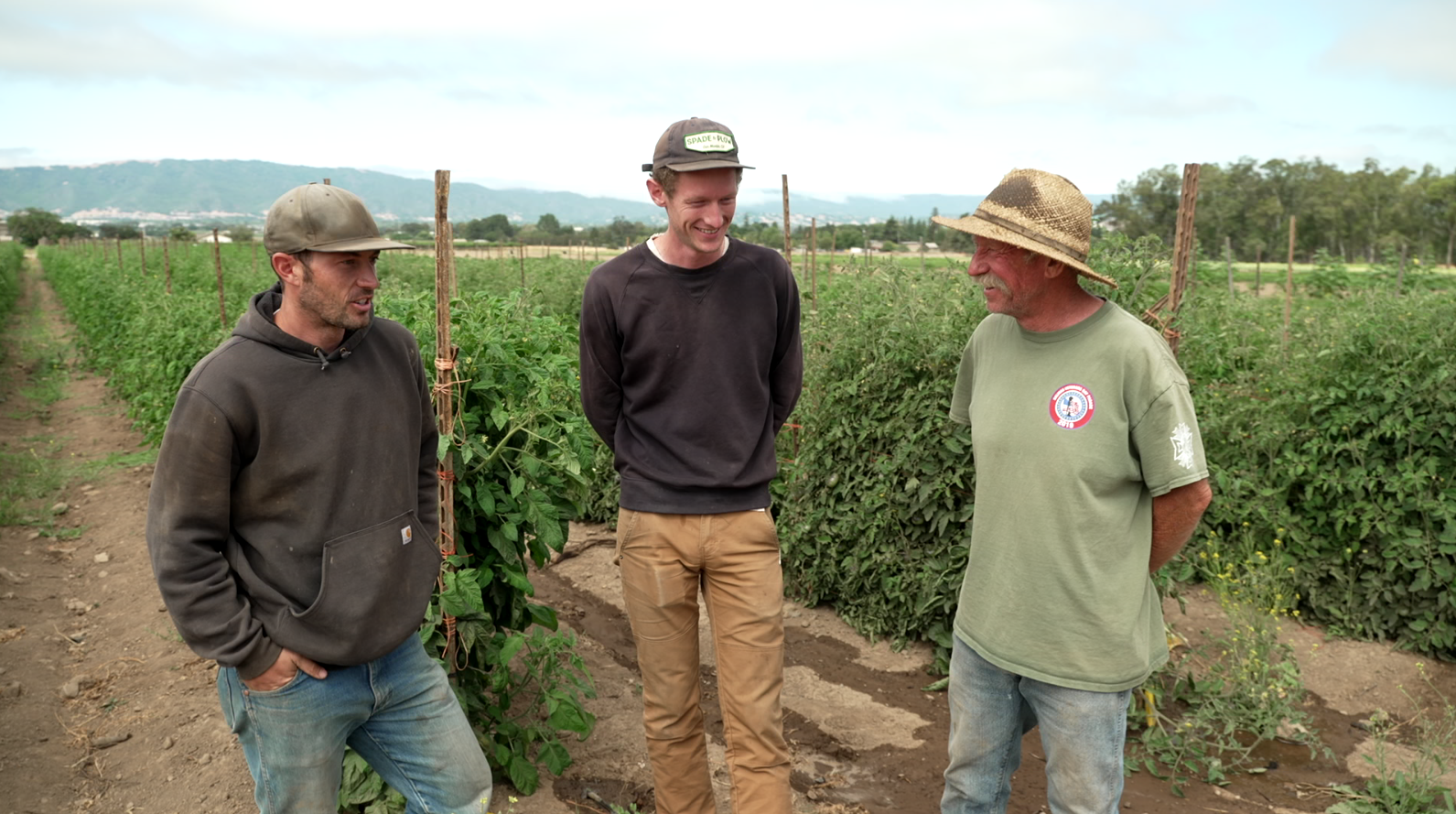In this image, three Caucasian men are standing in front of a vast farm field, with evenly spaced rows of stakes holding green plants in the background. The ground they stand on appears muddy and wet. The man on the far right is older, characterized by a gray mustache and a light green t-shirt with a symbol, paired with jeans and a farmer’s hat. The middle man, who is younger, wears beige Carhartt pants with a dark black sweatshirt and a green baseball cap. The third man on the left, also younger, is dressed in a brownish sweater and blue jeans, completing his look with a green hat. Two of them modestly have their hands behind their backs, while the middle man has his hands in his pockets. All three men, appearing cheerful and engaged in conversation, exhibit the traits of hardworking manual laborers. Behind them, a mix of bushes, trees, and mountainous terrain extends under a clear blue and white sky, indicating the vastness and natural beauty of their agricultural surroundings.